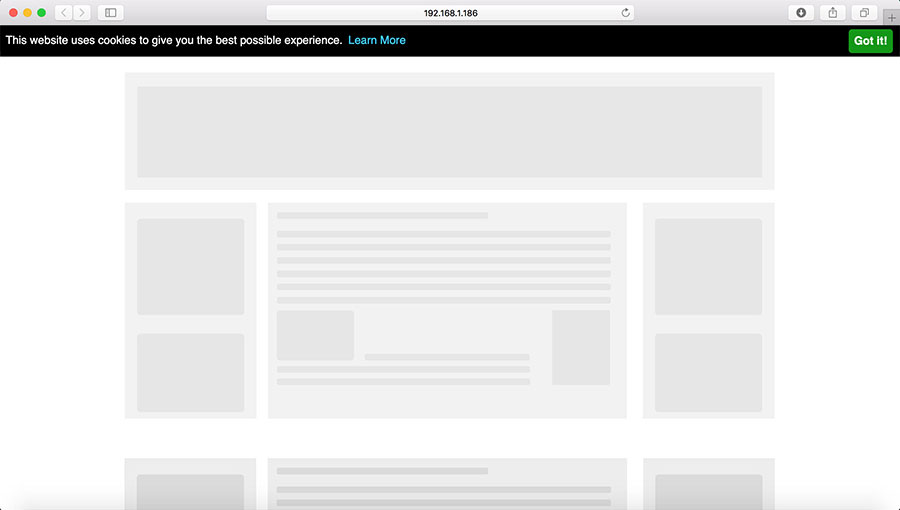The image depicts a detailed mock-up template for a web design interface. At the top, there is a gray bar with a series of controls. On the left side of this bar, there are three dots: a red dot, a yellow dot, and a green dot. Next to these dots is a cluster of icons, each contained within a white square. These include an icon with a left arrow, a white square with a right arrow, and an icon representing a webpage in gray.

In the center of the top bar is a URL input field displaying "192.168.1.186" in dark black lettering, indicating an IP address. To the right of the URL bar, there is a reload button. At the top right corner, there are three white background squares. The first square on the left contains a gray circle with a white down arrow. The second square features a gray square with a gray up arrow. The far right square displays two overlapping squares with a gray plus sign in the upper right corner.

Below this, there is a full-width black bar with white text that reads, "This website uses cookies to give you the best possible experience." To the right of this text, in blue letters, it says "Learn more." On the far right end of this bar, there is a green button with white text that reads "Got it!" 

Underneath this notification, the mock-up showcases a structured layout of placeholder content. At the top, there is a large rectangular space representing the banner area. Adjacent to it, the left column includes three image placeholders, and the right column also has three similar image areas. In the center, there are two text windows with gray lines denoting where text would be placed. The overall design presents a clean, organized framework for a potential webpage.